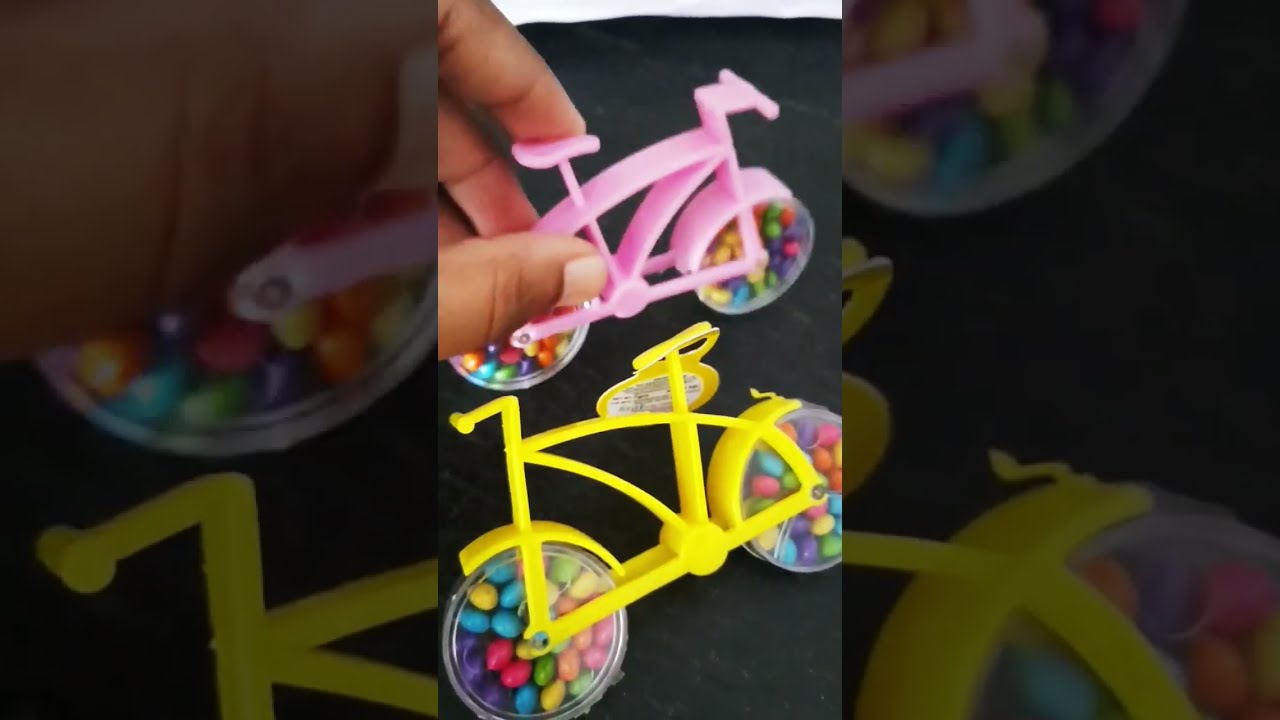The photograph showcases two small toy bicycles designed as candy holders, ideal for Easter baskets. One bike is yellow while the other is pink, each with clear plastic wheels filled with vibrant, pastel-colored candies reminiscent of M&Ms or gumdrops in shades of blue, pink, purple, green, and yellow. The candy-filled wheels are a delightful feature, with a black man's hand playfully turning the wheels of the pink bicycle. The bikes have flat plastic frames with curved seats and posts, adding to the whimsical design. The image includes a full view of the bikes in the center, bordered by a blurred enlargement of the same scene, providing a closer look at the intricate candy details and enhancing the overall visual appeal.